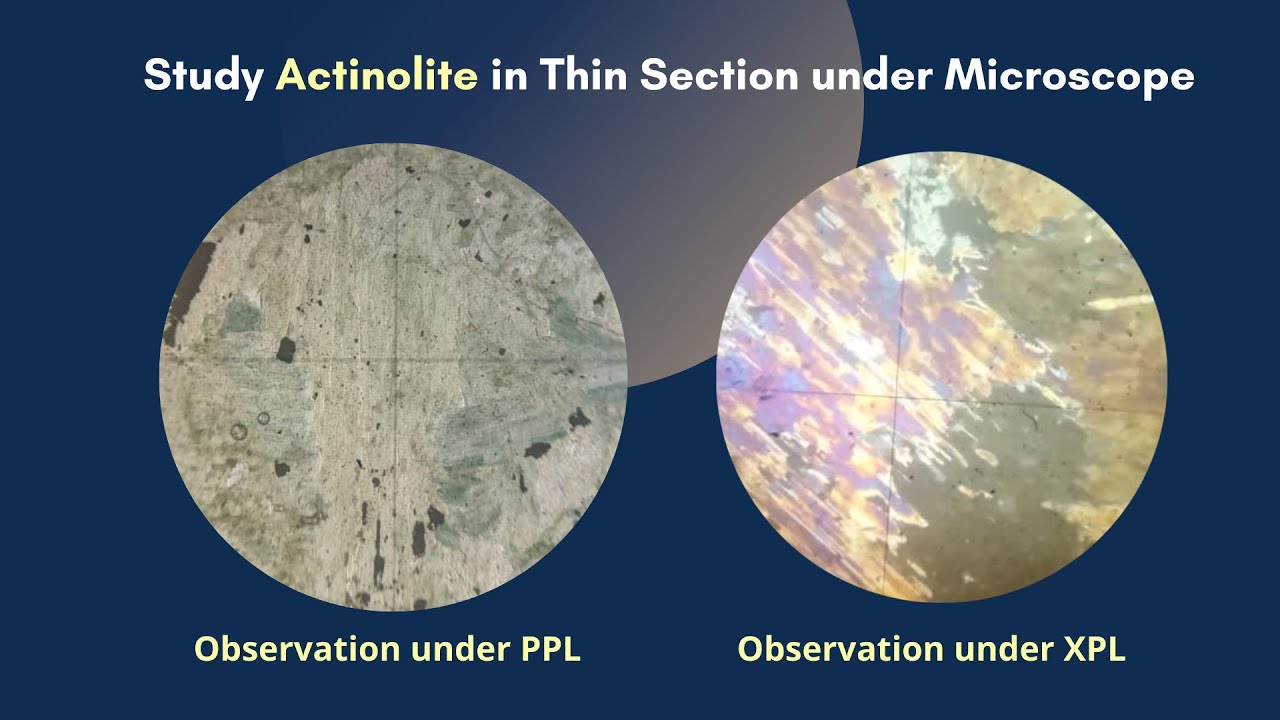The image features two circular microscope photographs with a blue backdrop, overlaid by white and yellow text. The header, “Study actinolite in thin section under microscope,” prominently features the word "actinolite" in yellow. The left circle, labeled "observation under PPL" in yellow text, displays a grayscale pattern with black speckles and a few bubbles. The right circle, labeled "observation under XPL" in yellow text, exhibits a vibrant, iridescent pattern with blues, browns, purples, oranges, and pinks, resembling a marbleized texture. This detailed illustration captures actinolite viewed under different polarizing light conditions, highlighting the contrast between the muted, speckled appearance under Plane-Polarized Light (PPL) and the strikingly colorful, streaked pattern under Cross-Polarized Light (XPL).